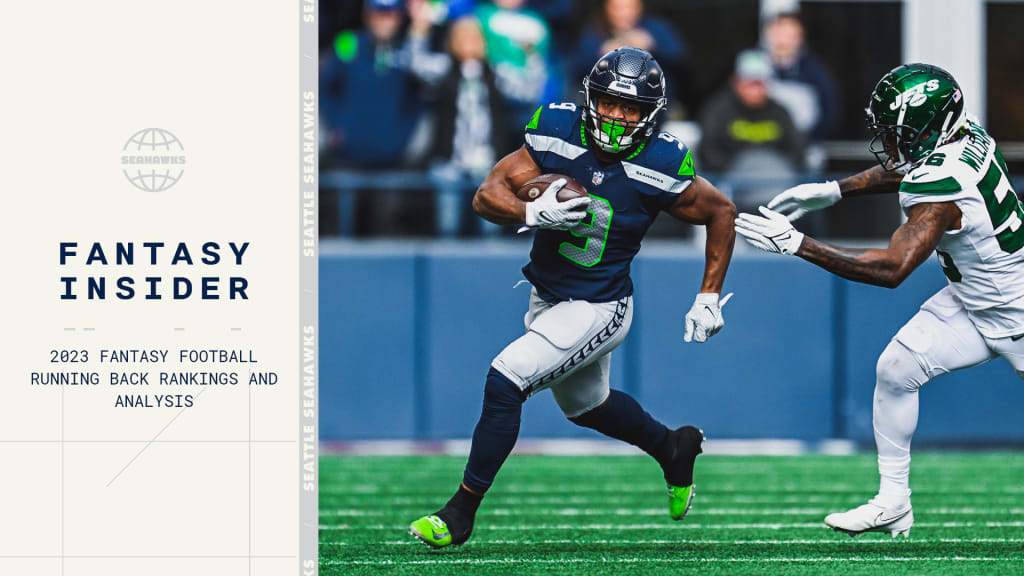The image prominently showcases two African-American football players from different teams in the midst of an intense play. The player in the foreground, wearing a blue jersey with a green "9" and white pants, is swiftly running with the football tucked in his right hand. His opponent, identifiable by his green helmet with "Jets" inscribed on it and donning green and white gear, is in hot pursuit, attempting to tackle him. Both players sport white gloves.

The backdrop features blurred spectators in the bleachers, emphasizing the action on the vividly green field marked with crisp white lines. On the left side of the image, bold text reads "Fantasy Insider," followed by "2023 Fantasy Football Running Back Rankings and Analysis." Above this text is a globe icon. A gray diagonal banner at the bottom left corner notes "Seattle Seahawks." The primary colors dominating the scene are blue, green, and white, with black text on a gray background for the Fantasy Insider section.